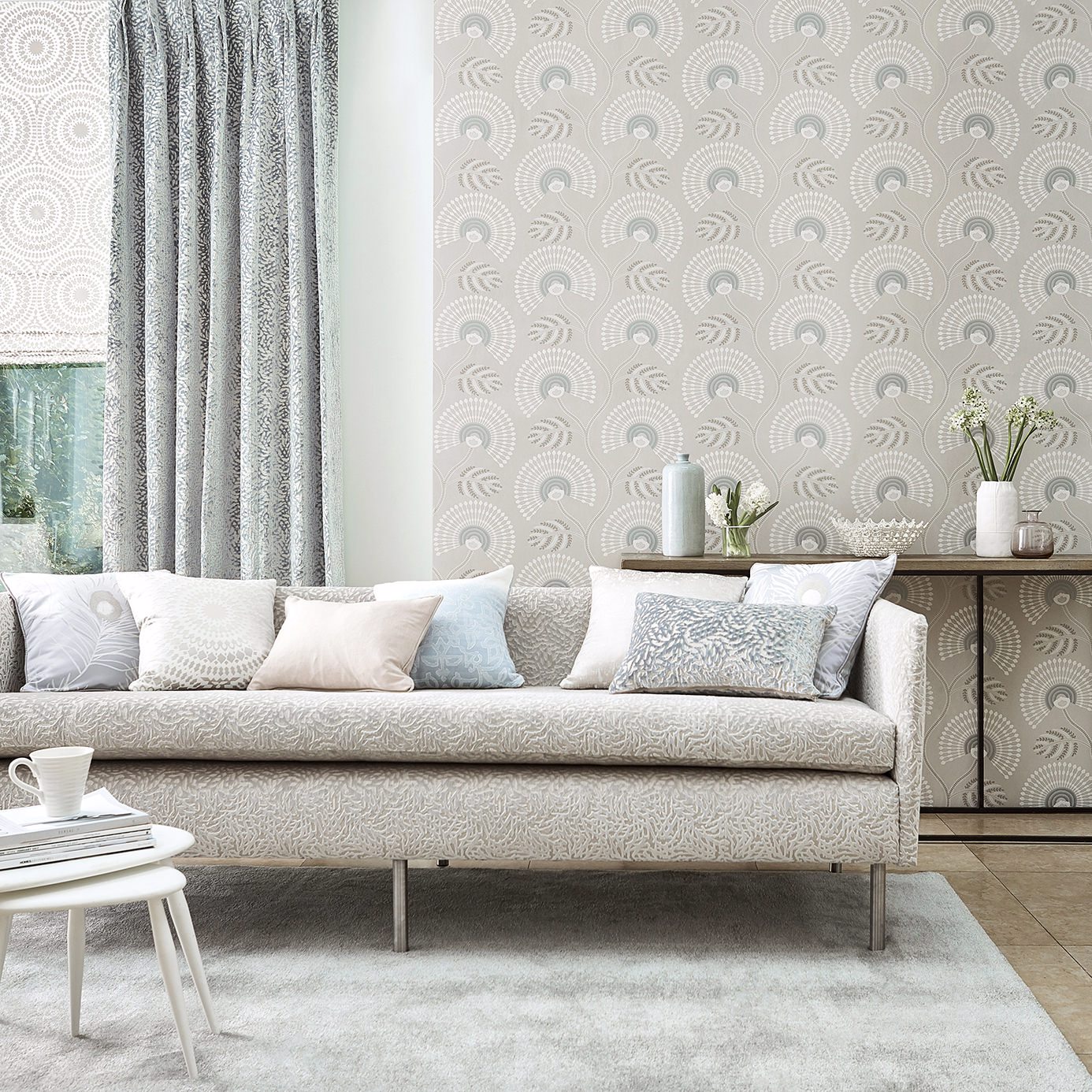The photograph showcases an elegant living room designed in tones of gray, white, and blue. Dominating the room is a long, comfortable-looking white couch with cylindrical chrome legs and several throw pillows, positioned centrally on a whitish gray carpet. In front of the couch sits a small white coffee table stacked with magazines and adorned with a white coffee cup. The backdrop features an exquisite wall covered in circular-patterned wallpaper with shades of blue, contributing to the room’s sophisticated aesthetic. Behind the couch, bluish-gray curtains frame a window, while a table behind the couch holds a vase of flowers and an empty white bowl, enhancing the space's decor. The room's overall look is cohesive and elegant, highlighted by the interplay of colors and textures.